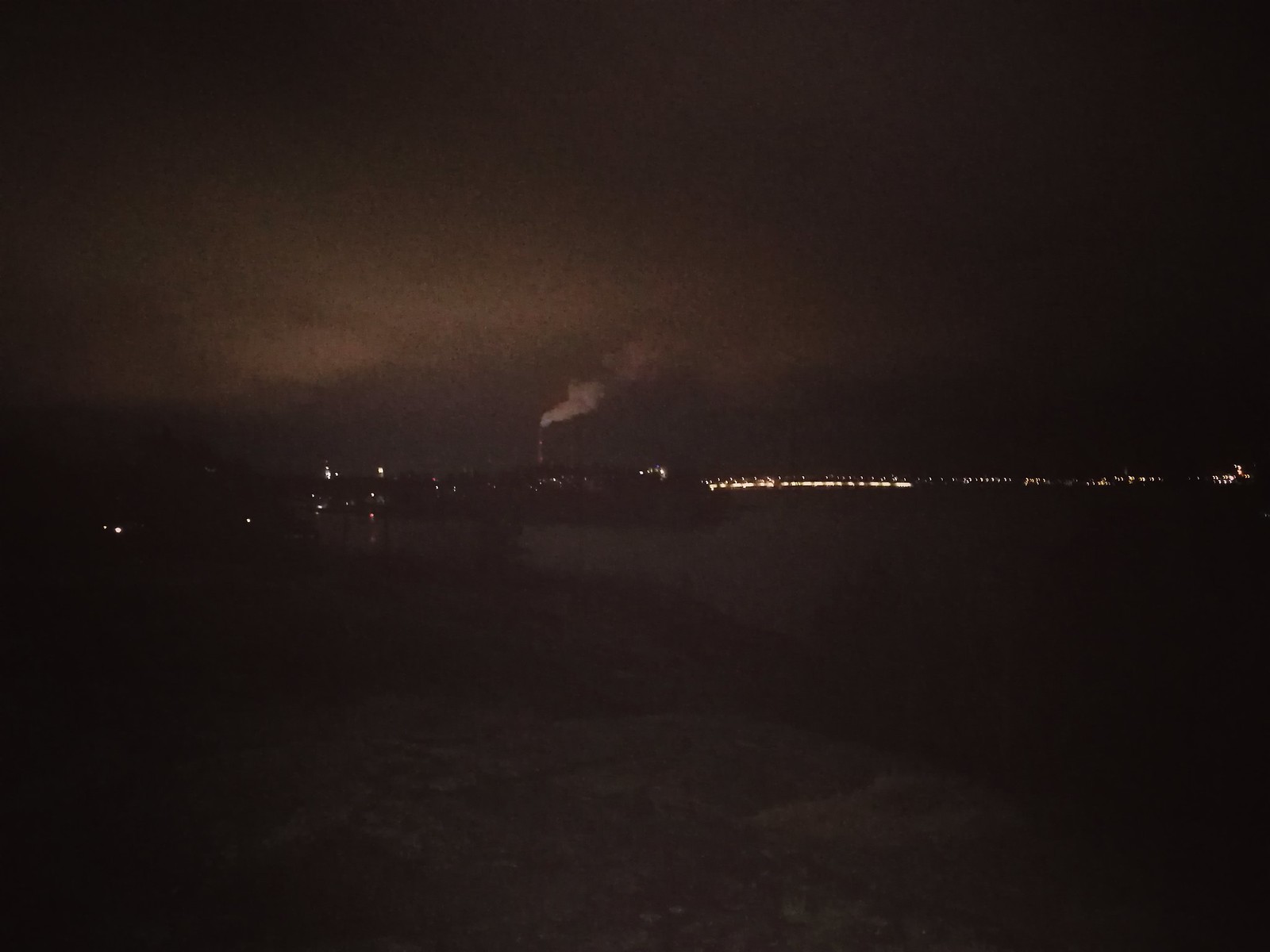A nighttime color photograph, likely taken from a rocky shoreline, depicts a bay filled with an array of lights stretching across the horizon. In the center-right, there is an evenly spaced string of lights that likely mark a low bridge crossing an inlet. To the left of this bridge, a factory with a smokestack is clearly visible, emitting white smoke drifting to the right. Further left, additional lights can be seen, illuminating clouds above in a light gray hue. The foreground is mostly dark, with faint hints of a shoreline or rocks, while any foliage present remains hard to see. The upper portion of the sky is uniformly black with no discernible features, making the overall image very dark and somewhat blurry, requiring careful observation to discern the details around the horizon.